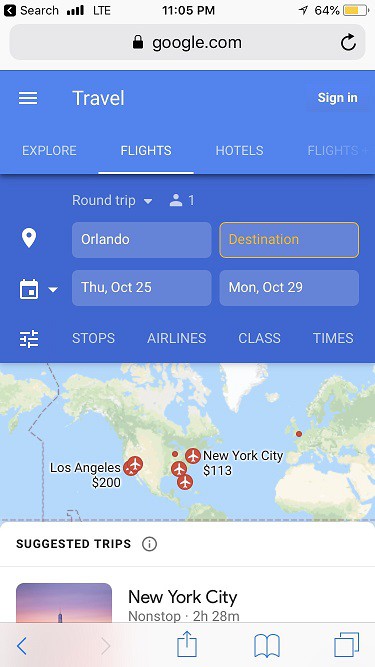This is a detailed screenshot from a smartphone displaying a search page on Google.com, specifically within the 'Travel' section. The phone has full signal bars with LTE connectivity, the time displayed is 11:05 PM, and the battery is at 64%.

At the top of the page, there is a search bar indicating "google.com," followed by a blue navigation band labeled "Travel," accompanied by a menu icon. To the right of "Travel," there is a "Sign In" option.

Below the blue navigation band, the options "Explore," "Flights," and "Hotels" are visible, with the beginning of the word "Flights" partially faded out. The next section features a darker blue box with the words "Round trip" in white letters, indicating the details of a planned trip. It mentions one traveler, departing from Orlando, with 'Destination' highlighted in orange within a blue box.

The travel dates are specified as "from Thursday, October 25th to Monday, October 29th." Further below, filter options for "Stops," "Airlines," "Class," and "Times" are available. Additionally, a map displays estimated travel costs with labels showing $200 for Los Angeles and $113 for New York City.